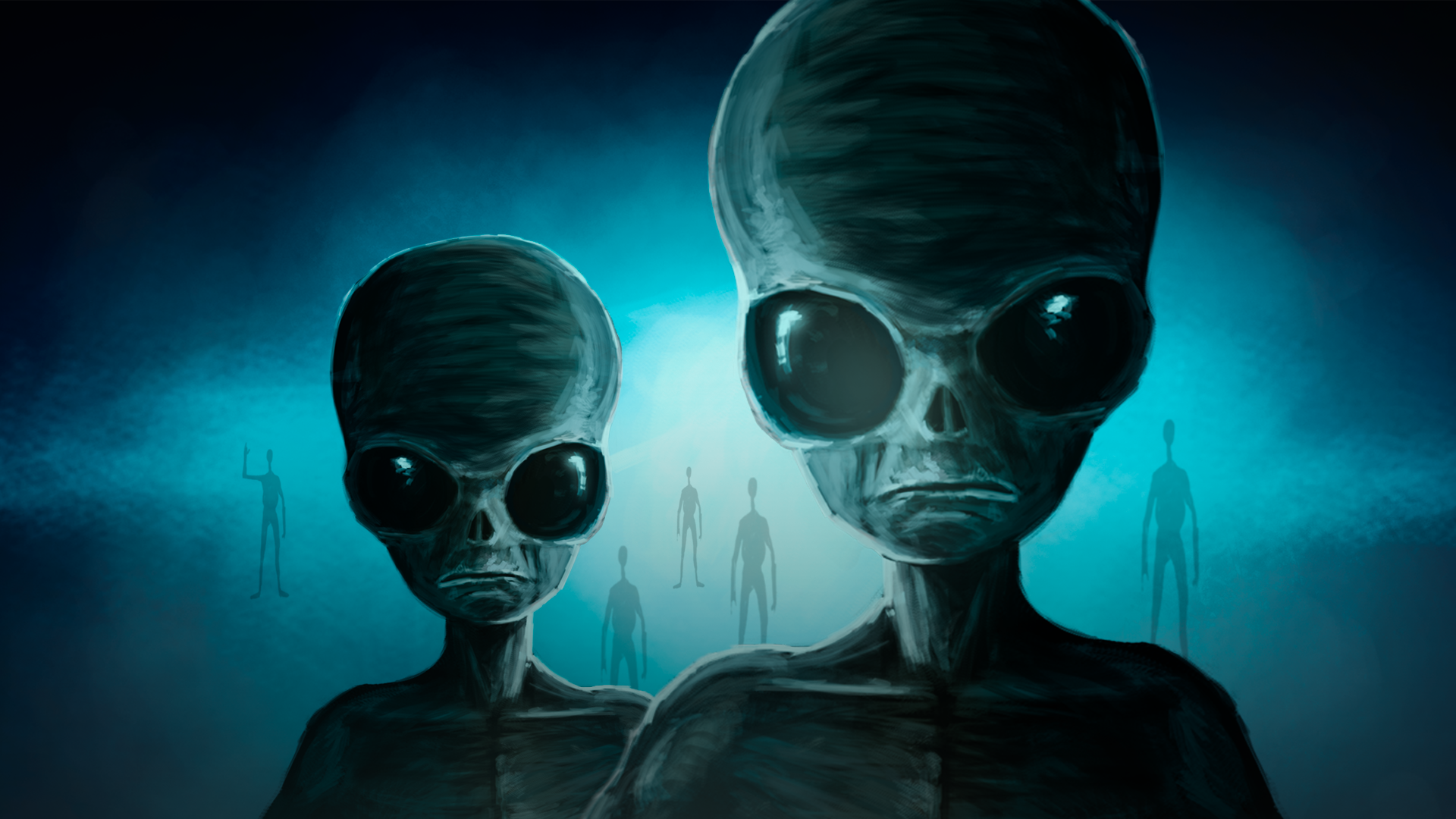In this eerie, dark painting, seven extraterrestrial figures emerge from a moody, blue-gray, smoky backdrop. At the forefront, two prominent aliens with large, domed heads and black, soulless eyes stare intensely at the viewer, their expressions stern and frowning. Their faces are marked by skeletal noses—mere slits—and their lips are thin, without visible teeth. These aliens have naked, skeletal-looking chests, and their gray skin is devoid of any hair. 

Behind them, five shadowy figures stand in a solid black background, with a bright blue light emanating from the center, casting an otherworldly glow. Among these figures, one on the left raises an arm in an L shape, while the others keep their arms at their sides. This scene, taken at twilight, exudes a creepy, fantasy-like ambiance, giving the impression of an alien invasion.